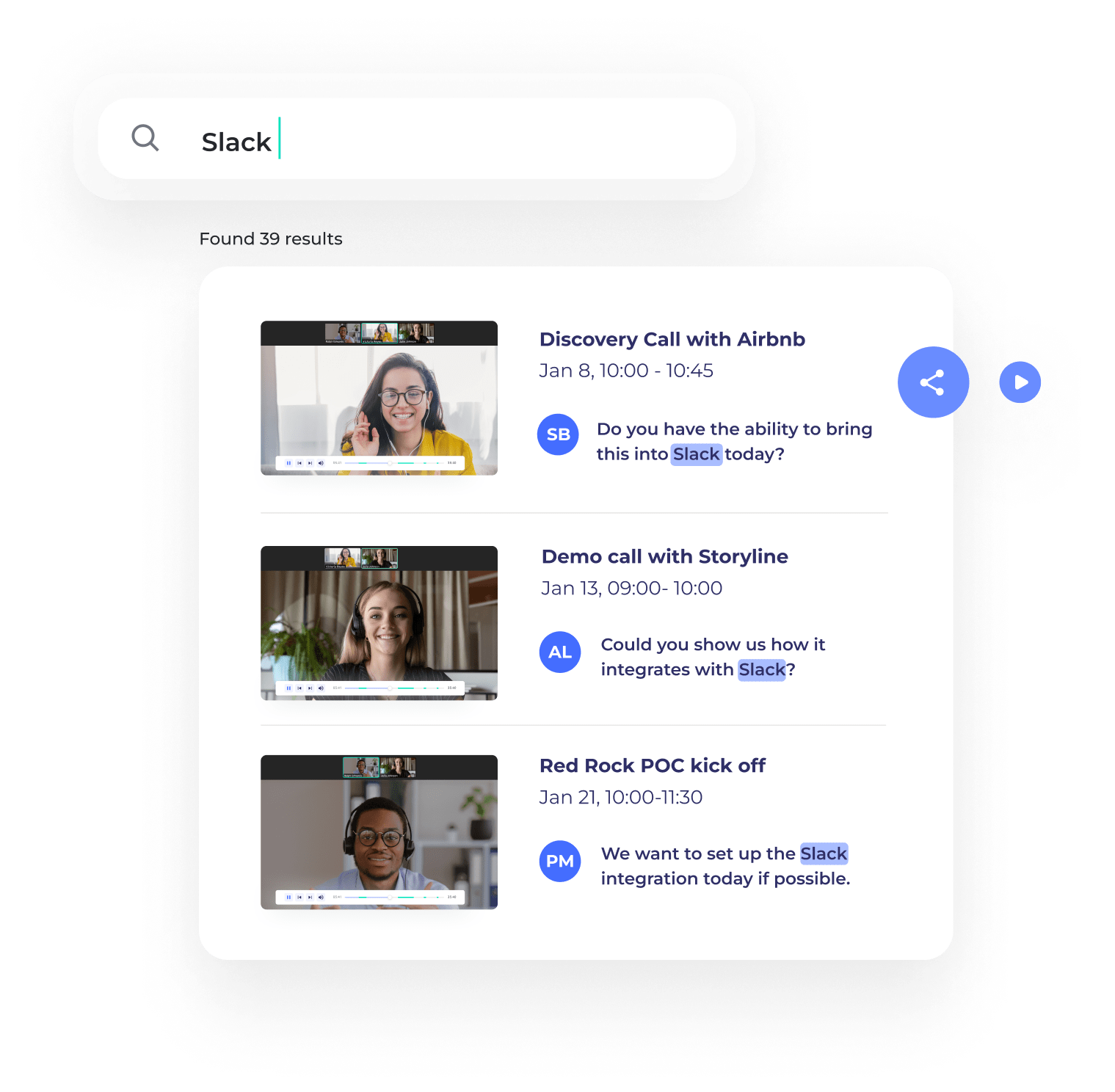This image is a screenshot of an interface displaying video thumbnails. At the top, a search box with rounded corners contains a magnifying glass icon on the left and the text "Slack" next to it. Just below the search box, a heading reads "Found 39 Results."

The main content area features a white box containing three video thumbnails. Accompanying each thumbnail on the right are the video's title, date and time, a blue circle with two letters inside it, and some descriptive text likely summarizing the video's content.

1. The top thumbnail shows a woman wearing a yellow top and glasses.
2. The middle thumbnail features a woman wearing headphones and a dark green t-shirt.
3. The bottom thumbnail displays a man wearing glasses, headphones, and a white shirt.

Also within this content box, a blue circle with a share icon is visible. On the far right edge of the screen, a smaller blue circle with a right-pointing triangle is present, likely indicating a navigation or play button.